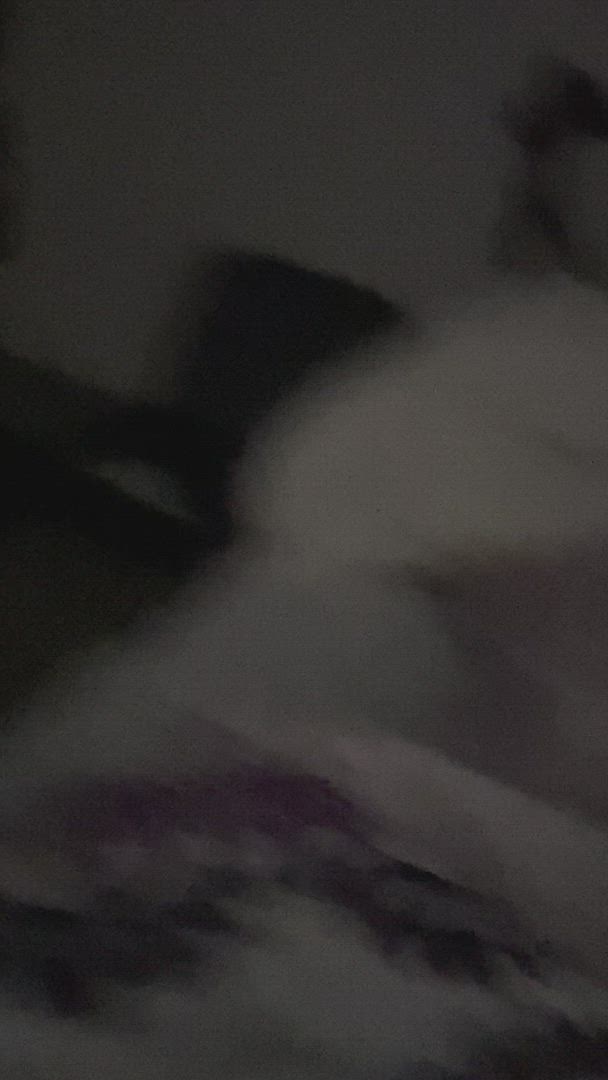This photograph captures an enigmatic and dimly lit scene, characterized by a significant amount of motion blur. In the shadowy composition, the barely discernable outline of a person appears amidst what seems to be a collection of bedding items, including pillows, a sham, and a blanket. The background features a wall, adding to the confined space's ambiance, suggesting a bedroom setting.

The blanket, while difficult to see clearly, appears to boast a floral design with violet-magenta flowers and dark green leaves scattered across a predominantly white fabric. The pillow sham, adding a touch of contrast to the scene, is a deeper off-white cream color. The interplay of shadows, motion, and muted light casts an air of mystery over the image, leaving much to the viewer's interpretation.